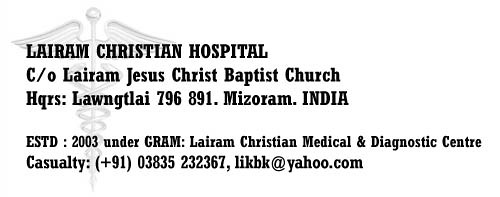The image appears to be a business card with a horizontal rectangular design and an off-white background. Prominently featured in bold, black text are the words "Laram Christian Hospital." Below this, it reads "C/O Laram Jesus Christ Baptist Church." The headquarters are specified as "Lawngtlai, 796891, Mizoram, India." The institution was established in 2003 under Graham and functions as the "Laram Christian Medical and Diagnostic Center." The word "Casualty" is also mentioned.

Embedded within the off-white background is a subtle watermark of the Caduceus symbol, which features a staff with wings and two snakes intertwined around it, rendered in light gray. Additionally, contact information is provided: a phone number "+91 03835232367" and an email address "likhk@yahoo.com."